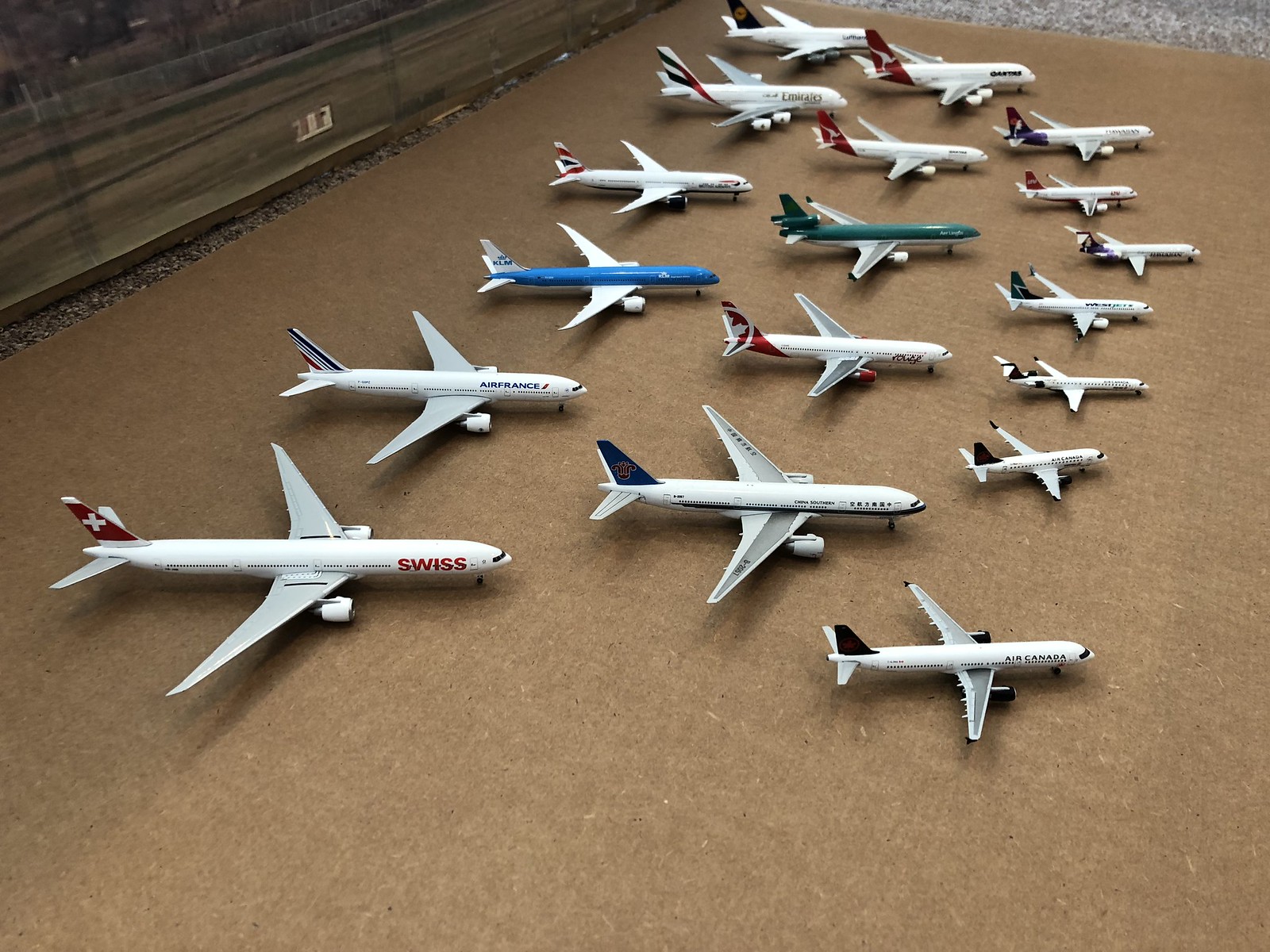The image showcases a meticulously arranged collection of miniature commercial jet planes, each adorned in various airline liveries. The planes, predominantly white with distinct airline-specific colors and markings, are organized in three rows against a tan or brown carpet background. The back row comprises six larger models featuring airlines like Swiss Airlines, identifiable by their white fuselage and red tails bearing the Swiss flag. Air France models are also present, marked by their striped tails in blue, white, and red. Another notable model represents Emirates, though it erroneously includes a Qatari flag depiction. The middle row consists of five similarly sized planes, while the front row displays the smallest models with a count of seven or eight. This setup suggests a careful and enthusiastic collector who enjoys the ability to view and appreciate the miniature planes, mimicking the orderly arrangement of aircraft at an airport.